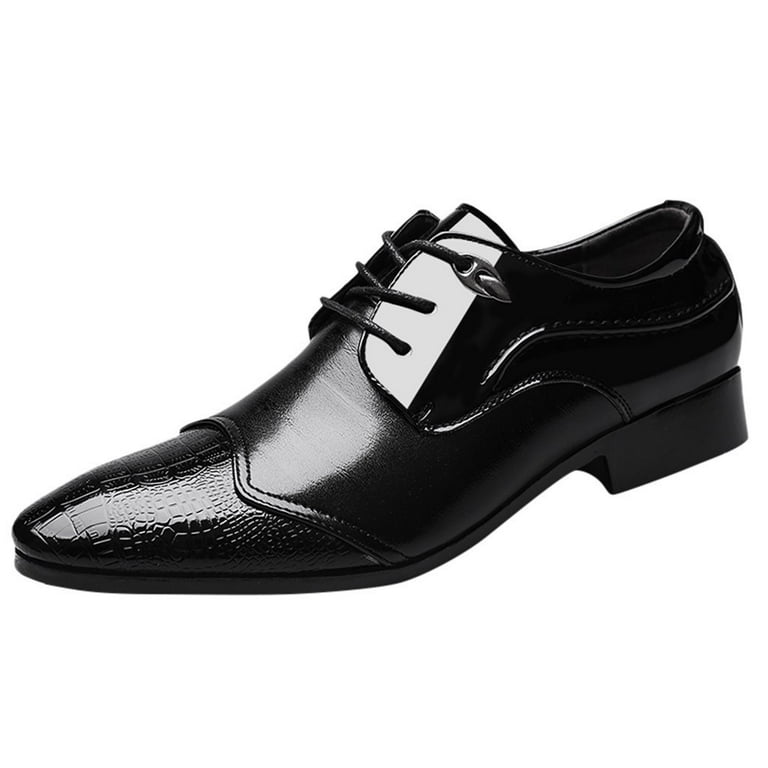This image features a polished leather dress shoe, likely male, presented in a computer-generated style against a white background. The shoe is oriented sideways, showcasing its left side profile with the toe pointing toward the lower left corner of the frame. The shoe comprises three distinct leather sections: the top part is a shiny patent leather that surrounds the laces, the middle section is a muted smooth leather, and the toe exhibits an alligator-like, reptilian texture. This all-black shoe has black laces that thread through three eyelets and incorporates a slight heel, approximately one inch in height, which is also shiny enough to reflect light. The double stitching on the toe, as well as the overall polished finish, highlights the detailed craftsmanship of the shoe.